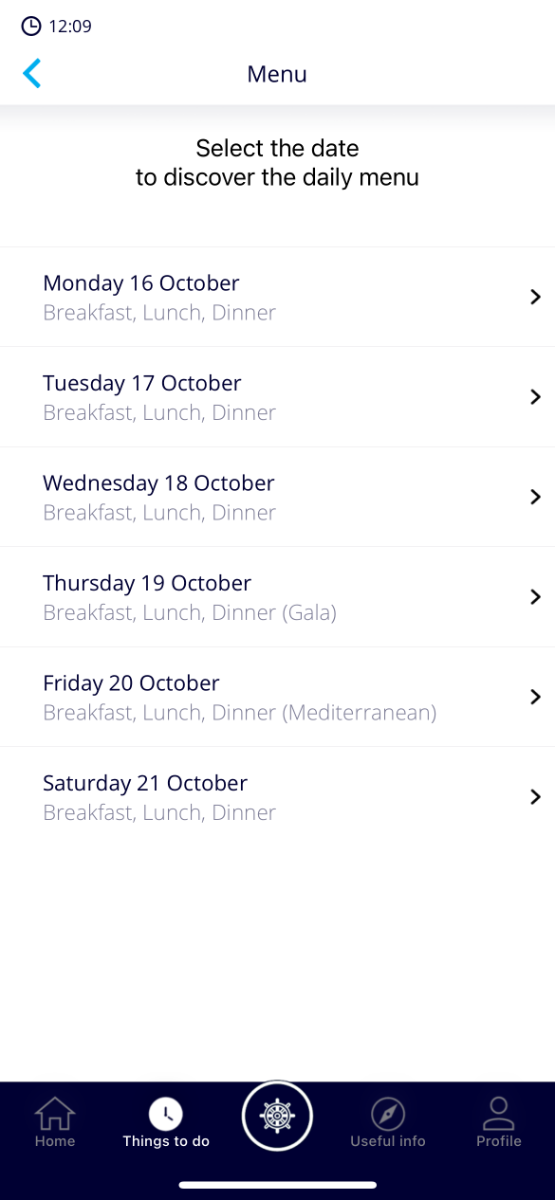The image is a screenshot from a cell phone displaying a menu selection screen. In the top left corner, the time reads 12:09. Dominating the middle section is the heading "Menu," followed by the instruction "Select the date to discover the daily menu."

Below this, a detailed list of dates and corresponding meal options is arranged in chronological order. Starting with Monday, October 16th, the menu options for "Breakfast," "Lunch," and "Dinner" are clearly listed. This format continues for the following days: 

- Tuesday, October 17th: "Breakfast," "Lunch," and "Dinner" in gray print.
- Wednesday, October 18th: "Breakfast," "Lunch," and "Dinner" in gray print.
- Thursday, October 19th: "Breakfast," "Lunch," "Dinner," and an additional option labeled "Gala."
- Friday, October 20th: "Breakfast," "Lunch," "Dinner," and an extra option marked "Mediterranean."
- Saturday, October 21st: "Breakfast," "Lunch," and "Dinner."

Each date entry ends with a right-pointing arrow. At the bottom of the screen, there is a black rectangle containing five white icons, arranged side by side, suggesting navigational or functional features of the app.